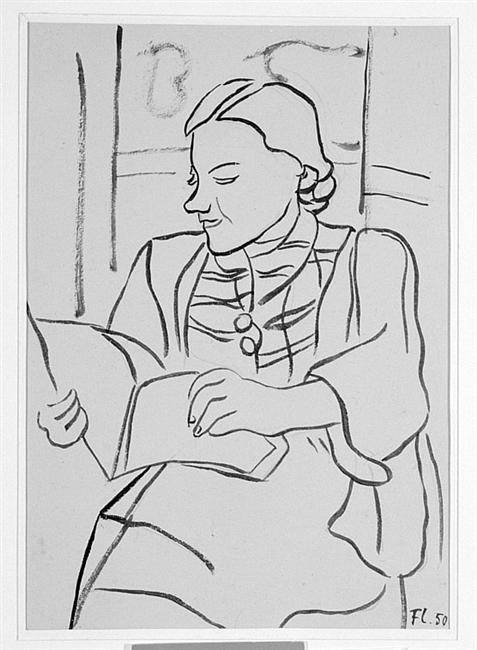This monochromatic black ink or charcoal drawing on white paper portrays a woman, aged between 30 and 50 years old, sitting and reading an open book. Her profile shows her large, pronounced nose and tightly tied back, longish hair. She is dressed in a long-sleeve outfit that covers her legs and her hands are visible. The central figure is meticulously detailed, holding a book and sitting slightly off-center. In the backdrop, there's a hint of a doorway or window, adding depth to the scene. At the bottom left corner, the text "FL50" is visible, likely the artist's signature. The overall impression of the artwork is that it might belong to a personal portfolio, perhaps reflecting an 18th or 17th-century setting based on the woman's attire and the archaic ambiance.